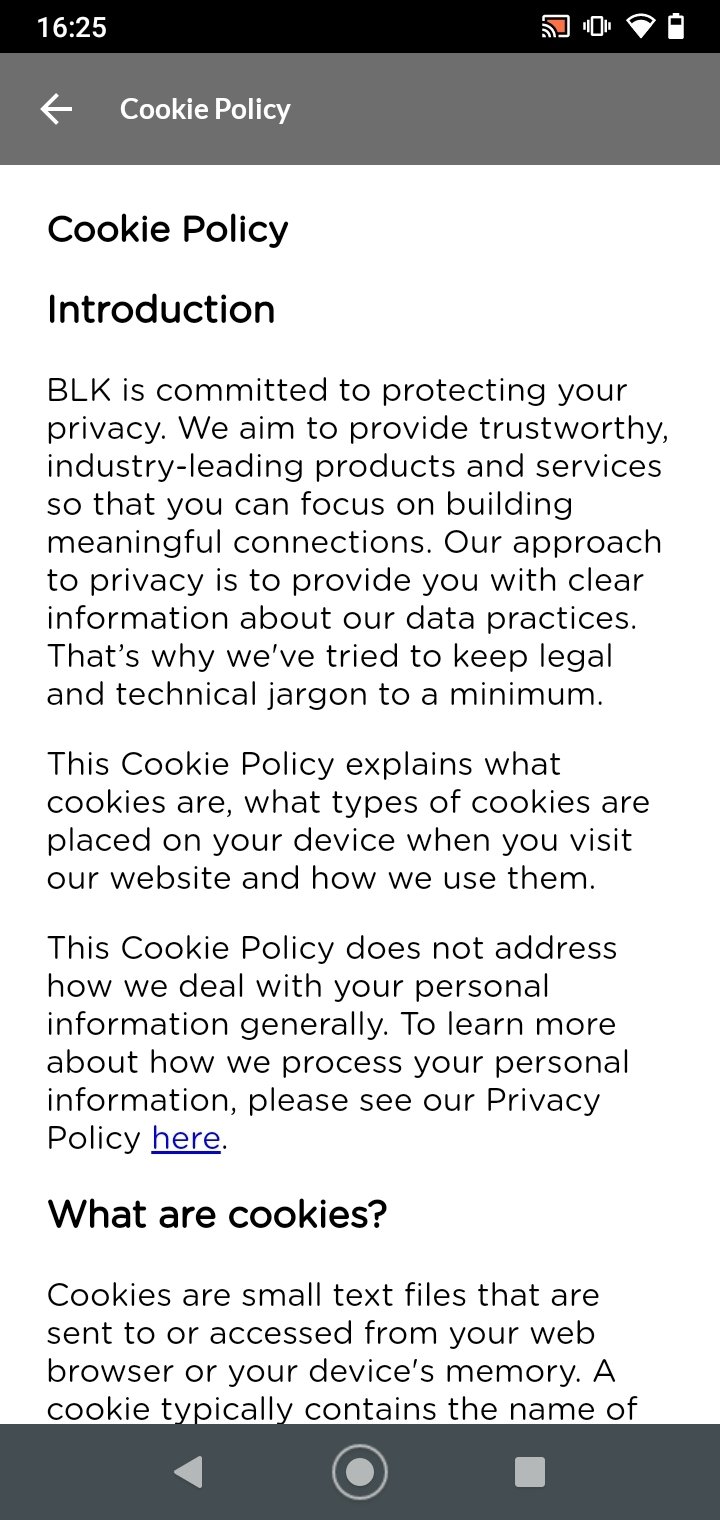**Descriptive Caption:**

The image features a white background with the text "1625 Cookie Policy" and an arrow pointing to the left, indicating the introduction to the cookie policy. It outlines BLK's commitment to protecting user privacy and their goal to offer reliable, industry-leading products and services to foster meaningful connections. The text emphasizes their approach to transparency by minimizing legal and technical jargon. 

The policy delineates the nature of cookies, detailing the types placed on user devices and their usage during website visits. It clarifies that the cookie policy specifically addresses cookies and does not cover broader personal information handling, directing users to the privacy policy for comprehensive information.

Highlighted in blue is the section titled "What are Cookies," explaining that cookies are small text files sent to or accessed from a user’s web browser or device memory. The visual elements include a black bar with symbols: a left-facing triangle, a circle, and a square.